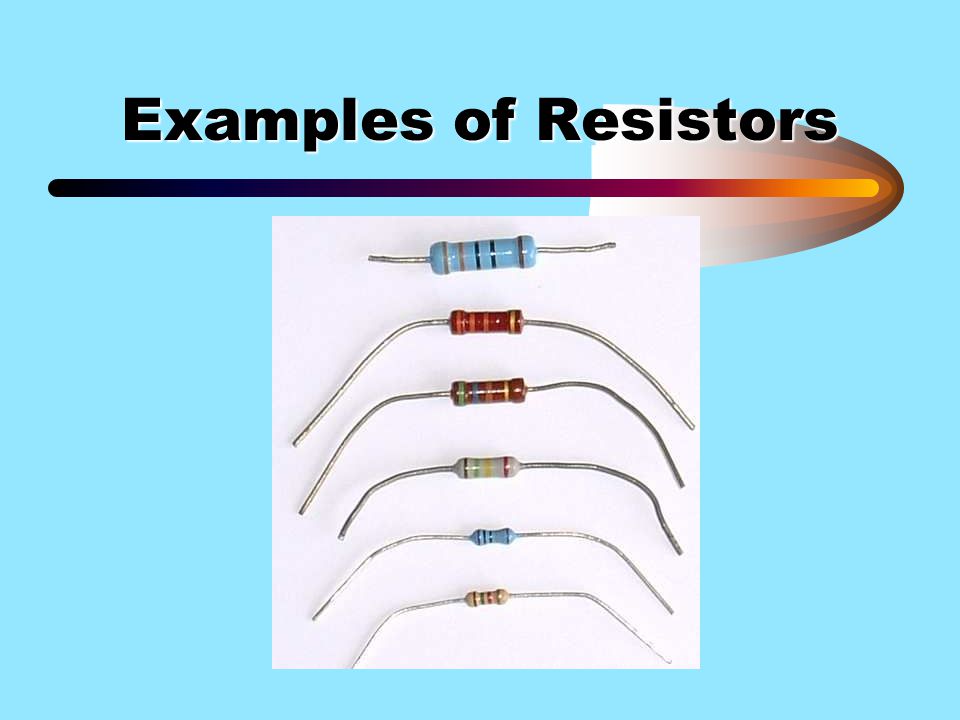**Poster Title: Examples of Resistors**

The poster, ideal for instructional use, features a light robin's-egg blue background. At the top of the poster, in large black text, is the title "Examples of Resistors." Below this title is a decorative line that transitions smoothly from black on the left, to blue, purple, brown, red, and orange on the right side.

Central to the poster is a white rectangle, slightly taller than it is wide, where the resistors are displayed. The rectangle houses six vertically stacked resistors with small spaces between them, each fitted with metallic wires extending from both ends.

From top to bottom, the resistors are as follows:
1. A blue resistor featuring gray, black, and brown stripes.
2. A red resistor with orange and yellow stripes.
3. A brown resistor adorned with green, blue, orange, and yellow stripes.
4. A solid white resistor.
5. Another blue resistor, similar to the top one.
6. A final white resistor, distinguishable from the fourth by slightly different tones and potential markings.